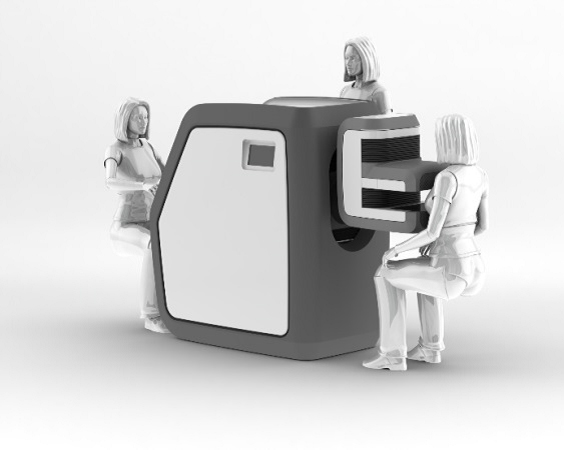The image depicts a stark white background showcasing three robotic, porcelain white female figures interacting with a large, dark gray, and cumbersome machine. The setting exudes a clinical and futuristic aesthetic, with the machine resembling a cross between an advanced medical device, possibly a mammogram or MRI machine, and an intricate model or prototype. The three robotic figures, devoid of distinct facial features, are positioned in varying postures that imply engagement with the device. 

One figure, akin to a squatting position, is butted up close to the machine, with its upper body pressed against an extension of the device that runs from her collarbone to below her bust line. Another figure stands behind the machine as if observing or overseeing the process. This figure's upper body is visible, suggesting she might be standing on an elevated platform, looking over the machine. The third figure is positioned on the far side, partially obscured by the device, and seems to be mimicking either a sitting or squatting posture. All three figures and the machine are rendered in grayscale tones, contributing to the scene's overall robotic and sterile ambiance.